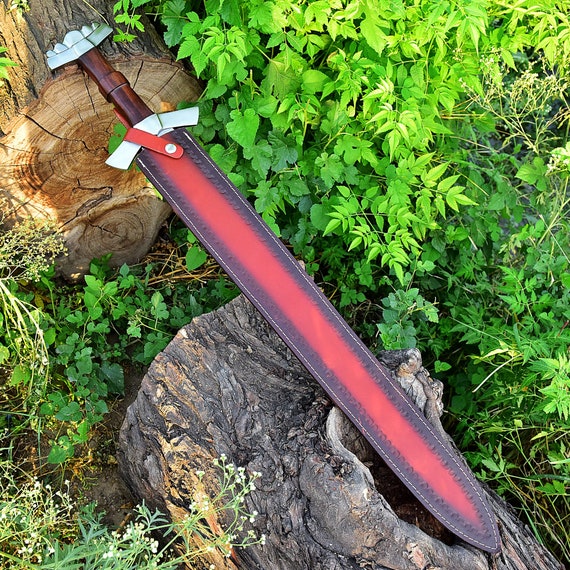The image displays an outdoor scene abundant with green foliage, various plants, grass, and dirt. At the center of the composition, there are two thick tree trunks laid diagonally, intersecting each other—one extending from the top left and the other from the bottom right. Between these trunks rests an ornate sword enclosed in a scabbard. The scabbard is predominantly dark brown leather with white stitching, featuring a striking light red streak running its length. The sword itself has a silver guard and a dark brown wooden handle with a circular detail in the middle, ending with a silver pommel. The scabbard is secured to the handle with a red strap, held by a white circle. The trunks, one light brown with multiple dark cracks and the other a darker gray, contrast with the lush green leaves that frame the scene, with some leaves appearing lighter due to sunlight. The camera angle suggests a top-down perspective, closely capturing the detailed textures of the logs, sword, and surrounding greenery.